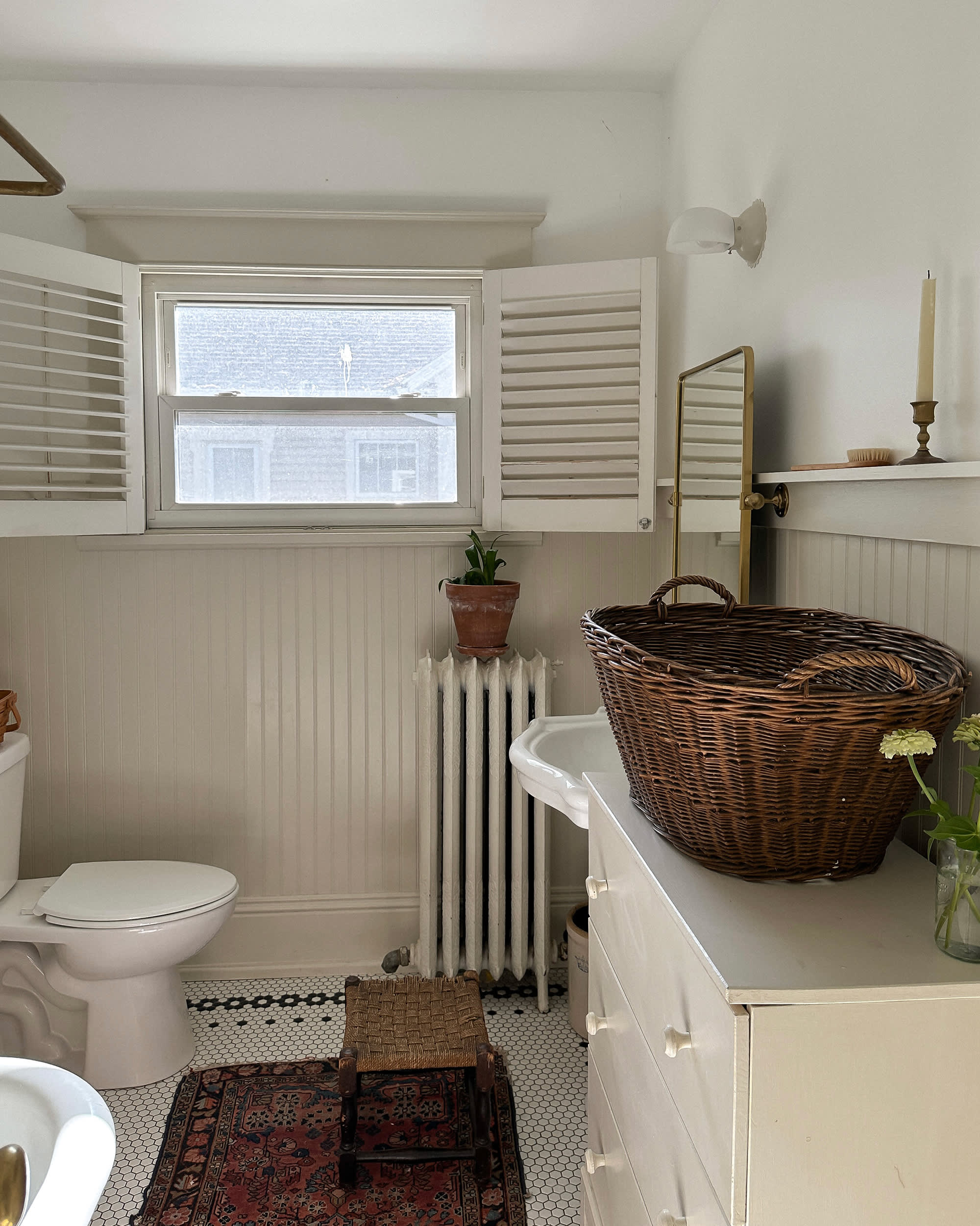This color photograph captures a beautifully designed bathroom primarily painted in white, giving it a clean and serene atmosphere. The backdrop features a shiplap wall with a rectangular window flanked by open white shutters, allowing light to fill the space. In the bottom left corner, a modern toilet, with its lid closed, sits adjacent to a partial view of a white sink.

The floor is adorned with black and white hexagonal tiles, accented by an ornate rug in dark red and brown tones. Positioned on the rug is a small brown step stool with a wooden top. Near the left side of the image, a white radiator warms the room, topped with a terracotta pot holding a vibrant potted plant.

In the right corner, a white chest of drawers stands with a dark brown wicker basket on top. Also on the dresser is a small glass jar containing yellowish-white flowers. High up on the wall above the dresser is a ledge occupied by a candle and a brush, adding a touch of homeliness. A gold-trimmed mirror with a light above enhances the simplicity and elegance of the space. Overall, this bathroom exudes a cohesive blend of cleanliness, functionality, and charm through its meticulous details.